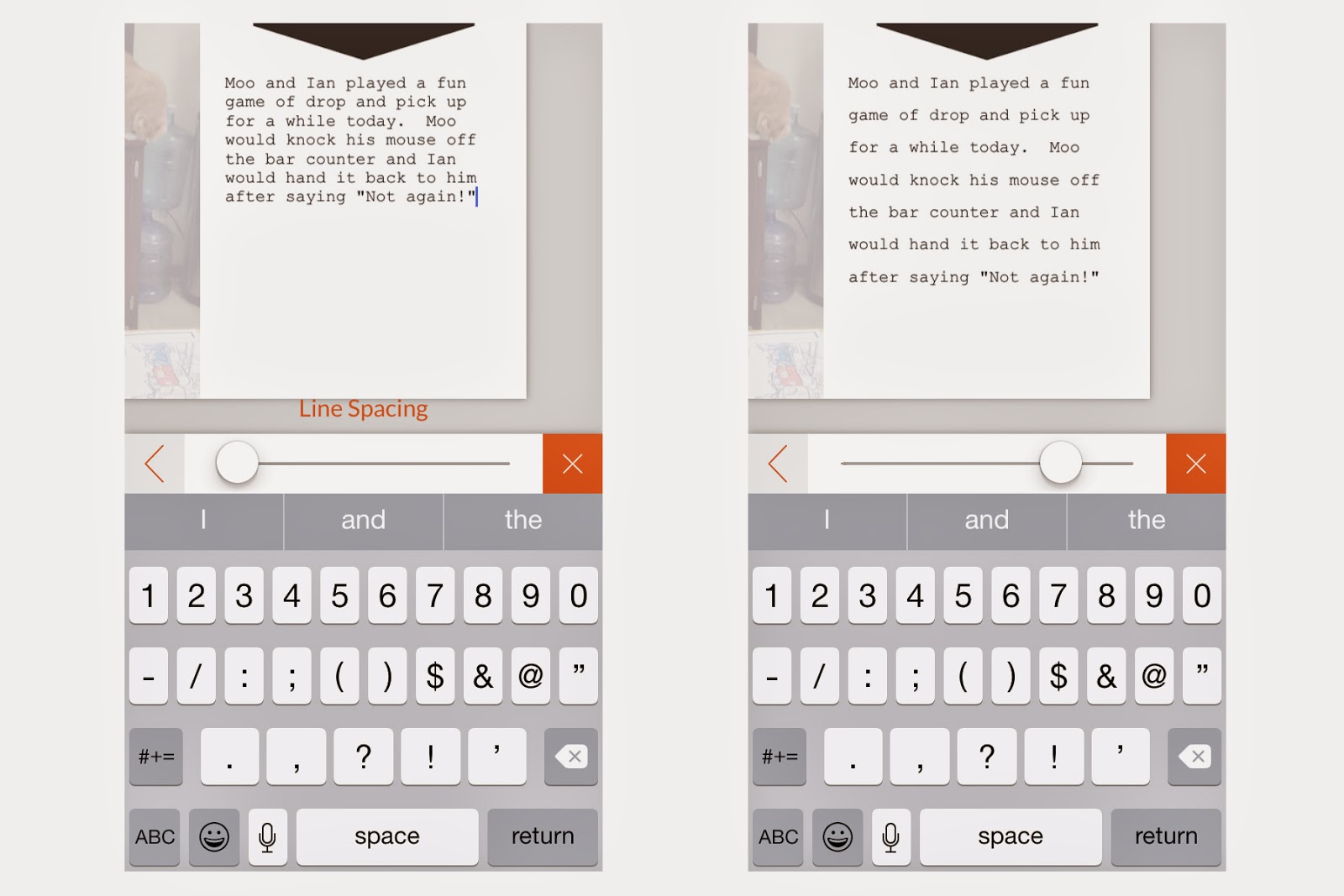The image depicts two cell phones placed side by side in a vertical orientation, resembling elongated rectangles. 

On the screens, there is a white page with black text at the top that reads, "Moo and Ian played a fun game of drop and pickup for a while today. Moo would knock his mouse off the bar counter and Ian would hand it back to him after saying 'Not again!'."

Below this text, an orange interface element labeled "Line Spacing" is visible. It includes a slider bar that can be adjusted back and forth. Currently, the slider is positioned all the way to the left. Accompanying this slider is a left-pointing arrow on its left side, and an orange box with a white "X" on its right side.

Further down the screen, there is a virtual keyboard set to its numeric layout, where the main keys are white with black numbers, while the secondary keys are gray.

On the second cell phone, the displayed text is identical but formatted differently, reflecting changes in line spacing. "Moo and Ian played a fun game of drop and pickup for a while today. Moo would knock his mouse off the bar counter and Ian would hand it back to him after saying 'Not again!'." differs from the first screen, as the lines of text are more spread out. The line spacing slider on this screen is moved more towards the right compared to the first phone, though not fully to the right side.